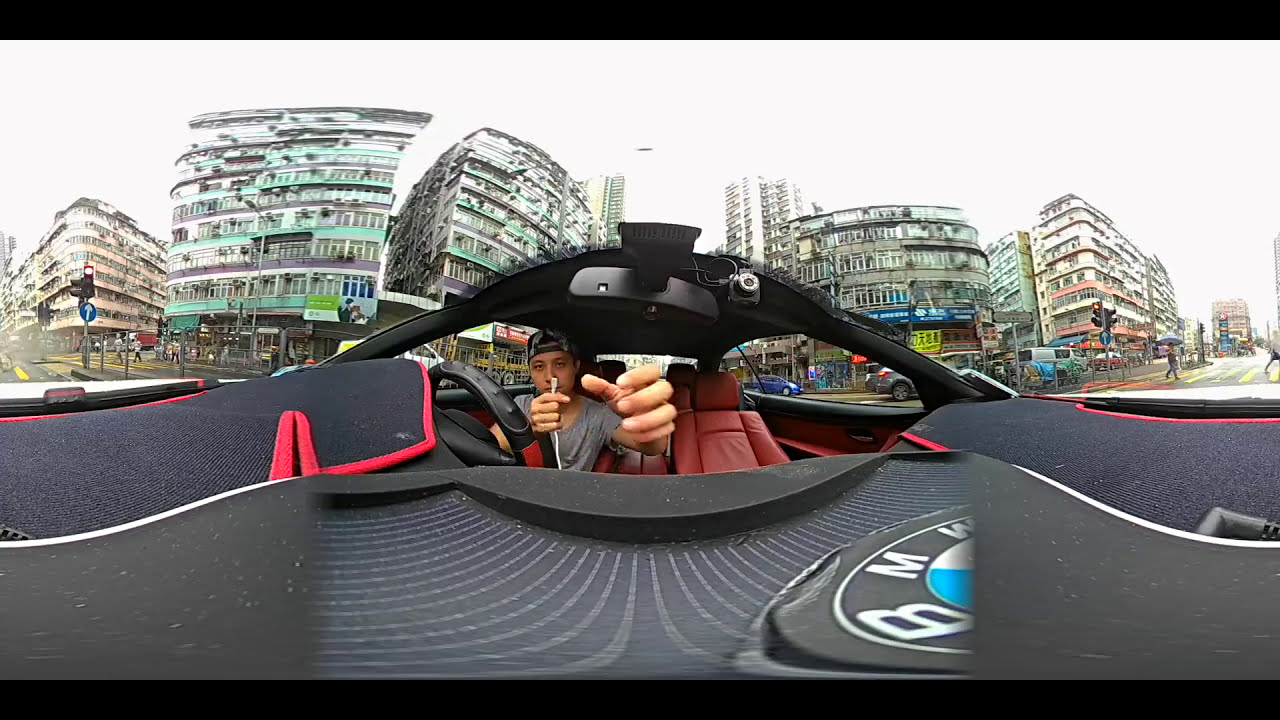The image depicts a man driving a sleek, black and red BMW sports car. The photo appears to be taken from a front-facing camera mounted on the hood, providing a clear view into the car's interior which features luxurious red leather seats. The driver, wearing a grey t-shirt and a backwards baseball cap, is positioned on the right side of the vehicle, possibly suggesting the car is in a country with right-hand driving. He is holding a white cable in one hand while stretching the other.

Surrounding the car, there is a bustling cityscape characterized by an array of tall residential or commercial buildings, some green and others white with red trim, typically found in an Asian country. These buildings line both sides of a long road filled with other cars and pedestrians. In the distance, multiple traffic lights are visible, all showing red signals. A sign post with a blue circular sign and a white upward-pointing arrow can be seen on the left. The sky above is overcast, casting a diffuse brightness over the scene, indicating it's daytime.